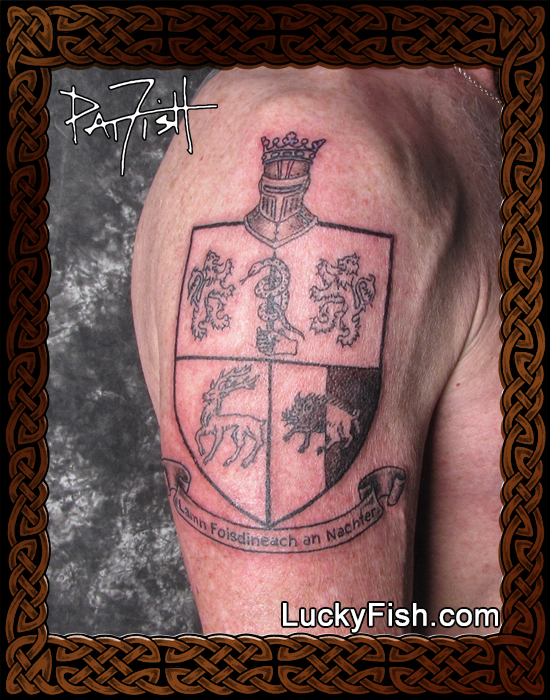The image depicts a close-up of a pale-skinned man's right shoulder and bicep area, showcasing a freshly done, intricately detailed tattoo. The skin appears slightly red and irritated, suggesting recent work. The tattoo is a coat of arms or crest shield featuring a knight's helmet adorned with a crown at the top. Inside the crest, there are two lions standing with their front legs raised, flanking a snake entwined around a sword in the center. The lower-left quadrant of the shield contains a deer or antelope with backward-curved horns, while the bottom right quadrant features a half-black, half-white boar or warthog. Beneath the crest, a banner bears the text "Lahnfosdinasanachter" or a similar foreign inscription. 

The photograph itself is set against a gray and white speckled background and is framed by a black border with a looped bronze design. The image bears the signature "Pat Fish" in an artistic white print in the upper left corner and the website "luckyfish.com" in white text in the lower right corner of the photograph.